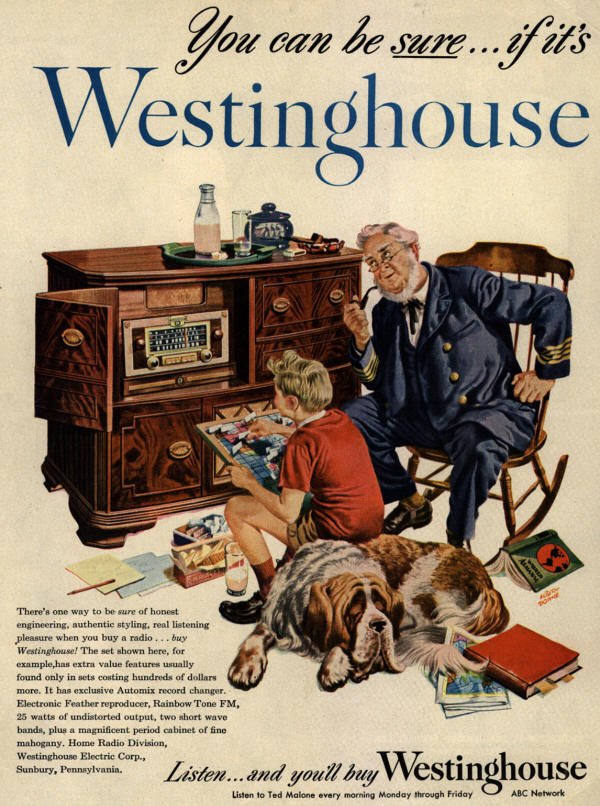This vintage advertisement, rendered in a classic illustrative style typical of old-school magazine prints, showcases a cozy indoor scene centered around a Westinghouse radio. The scene features an elderly man with a gray beard and glasses, dressed in a formal sailor-like captain's suit and bow tie, smoking a pipe, and sitting in an antique wooden rocking chair. Next to him, a young boy, about ten years old, with blonde hair, red t-shirt, brown shorts, red socks, and black shoes, is sitting on a large St. Bernard dog. The boy appears to be engaged in a puzzle or board game.

The focal point of the room is a solid cherry wood entertainment console against the wall. The console dresser has drawers and an open compartment revealing a Westinghouse radio. On top of the console sits a tray with a bottle, a glass of water, an ashtray, matches, and a small pot. Scattered on the floor are hardcover books, papers, a pencil or pen, and a glass of milk next to the boy.

The ad’s text includes several key statements: "You can be sure… if it’s Westinghouse," with "sure" underlined, and "Listen and you'll buy Westinghouse." Additional small print details the radio's premium features: "There's one way to be sure of honest engineering, authentic styling, real listening pleasure when you buy a radio by Westinghouse. The set shown above, for example, has extra value features usually found only in sets costing hundreds of dollars more. It has an exclusive auto-mix record changer, electronic feather reproducer, rainbow tone FM, 25 watts of undistorted output, two short wave bands, plus a magnificent period cabinet of fine mahogany." This is followed by "Westinghouse Electric Corp, Salisbury, Pennsylvania," and a reminder to "listen to Ted Malone every morning, Monday through Friday, ABC network."

This detailed illustration effectively communicates the warmth and quality associated with owning a Westinghouse radio, promising both aesthetic appeal and superior engineering.